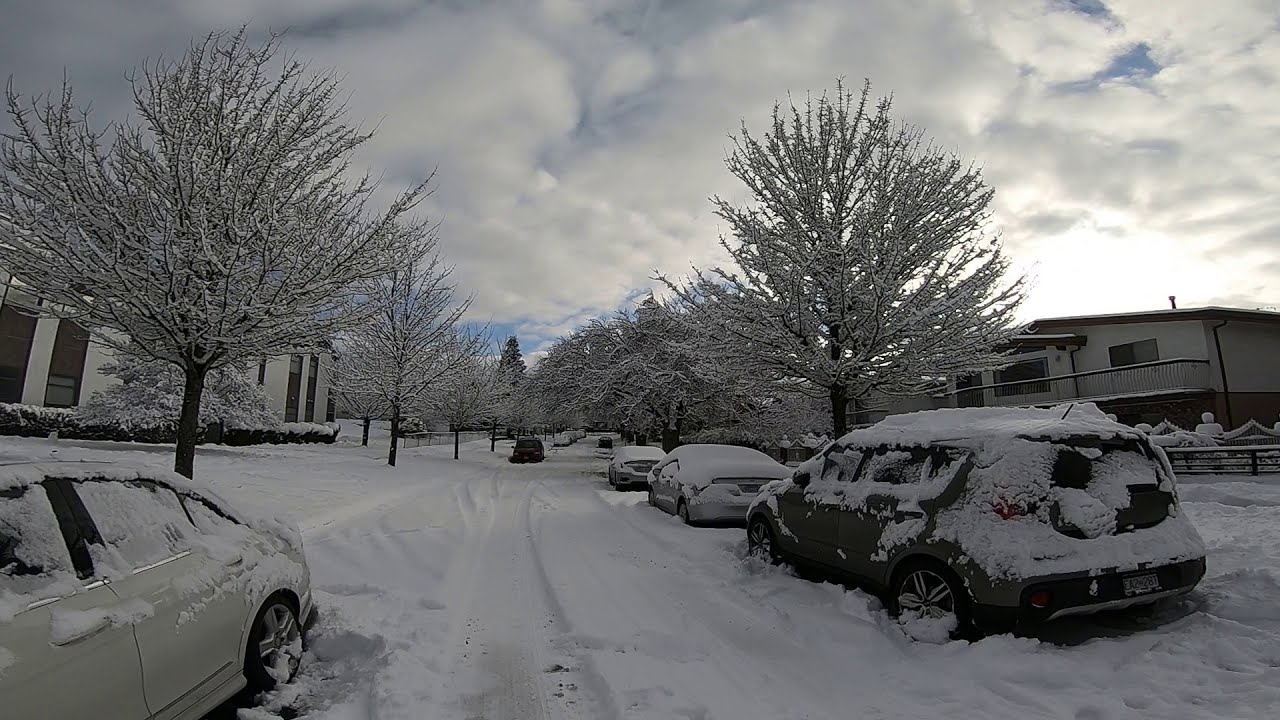The photograph captures a serene, wintry suburban street scene as daylight transitions into the evening. The viewer stands in the center of an untouched snow-covered road, surrounded by a quiet neighborhood blanketed in freshly fallen snow. To the left, a single white car sits parked and fully covered in snow at the lower corner of the image. On the right, three vehicles—beginning with a gray SUV, followed by a lighter gray or silver car, with another car further ahead—all are similarly shrouded in snow. Trees, stripped of their leaves but adorned in frosted branches, line both sides of the street, standing about 30 feet tall. Behind these trees, a mixture of apartment buildings and houses are visible, adding to the residential charm. Above, the sky is predominantly cloudy with streaks of blue, hinting at a hazy sunset peeking through the clouds on the right-hand side, casting a gentle light over the picturesque scene. Tire tracks are the only disturbance in the otherwise pristine snow on the road, suggesting recent but minimal human activity. The scene is captured in color, emphasizing the photorealistic beauty of this tranquil winter landscape.